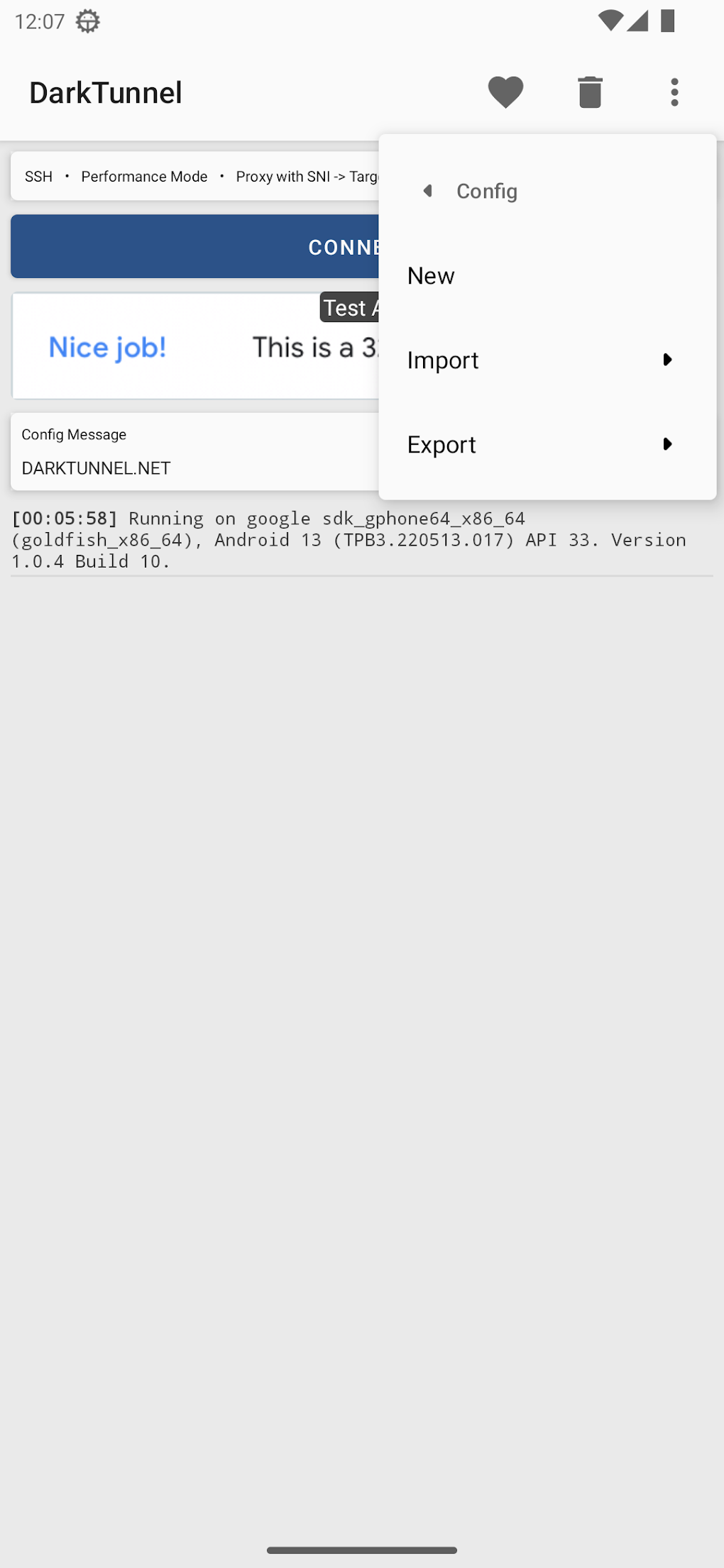Captured on a smartphone, this mobile screenshot has a predominantly light gray background and features a variety of elements that suggest it is a configuration page for a proxy setup. 

At the very top of the screen, the header bar displays the current time as 12:07 in the upper left corner. To the right, three gray icons are closely grouped together, followed by another three icons directly beneath them—a heart, a trash can, and three vertical dots.

In the top left corner of the banner, the screen identifies a section named "Dark Tunnel." A square pop-up box overlays part of the upper section, displaying options like “Config” with a left arrow, “New,” “Import” with a right arrow, and “Export” with a right arrow as well.

Beneath the overlaying pop-up, a partially visible blue header bar reads "Connect," with "C-O-N-N" clearly visible. To the left of this bottom bar, there is a tab labeled "Nice Job." Below this tab, the text reads "Config Message Dark Tunnel.net" with some very small Arial font underneath, which states, "Running on Google with some numbers, in parentheses, Goldfish//86/64 Android 13."

An address bar then follows this, reading “Performance Mode Proxy with SNI,” indicating that this is indeed a configuration page for a proxy. At the bottom center of the screenshot, there is a short gray horizontal line, completing the detailed layout of the screen.